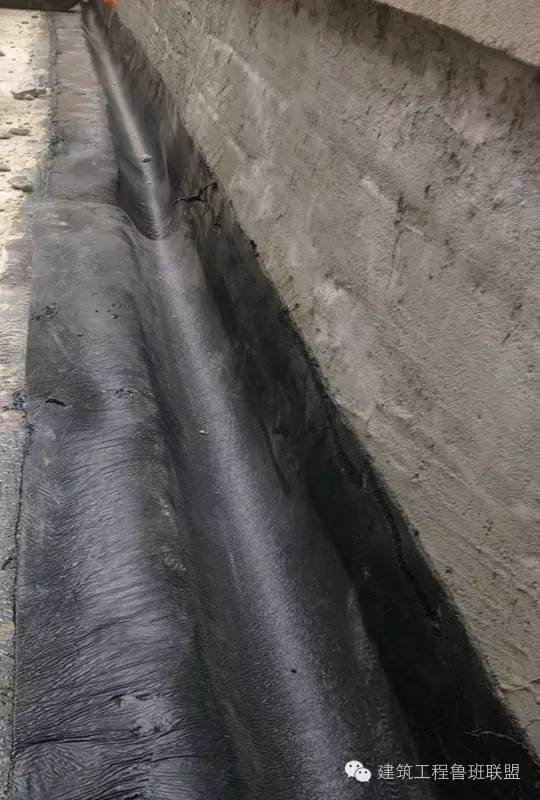In this image, a stark gray concrete surface dominates the frame, giving an impression of cold industrial simplicity. At the base of the image, an area coated in black tar stretches across, adding a contrasting dark element. On the bottom right, a series of inscriptions in an unfamiliar script, possibly Chinese, adds a mysterious cultural touch to the scene. Two prominent white circles punctuate the gray expanse, each marked with small black dots that could be interpreted as tiny ants. These circles are situated on the concrete, creating a curious focal point. The top of the image features a slight elevation, or 'lip', where the surface becomes level, separating into two distinct sections. The right-side lip is notably taller, framed by more gray concrete, creating a sense of asymmetry. In contrast, the lip on the left is lower and blends smoothly with the surrounding gray areas, while a darker patch on the right side hints at a possible shadow or stain, adding depth and texture to the image.